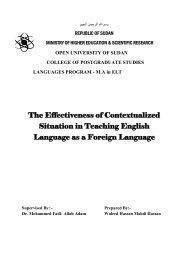This image features an academic document with a white background, displaying the title "The Effectiveness of Contextualized Situations in Teaching English Language as a Foreign Language" prominently in a bold black font. At the top, it reads "Republic of Sudan" followed by "Open University of Sudan," and "College of Postgraduate Studies Language Program." On the left side, there is a 3D-like hazard symbol composed of multiple lines. The text at the bottom is faint and blurry, indicating that the document was proposed by an unnamed individual and supervised by Dr. Mohammed Falk. The overall text is small and challenging to read, suggesting this image might be from a dissertation or an academic article.